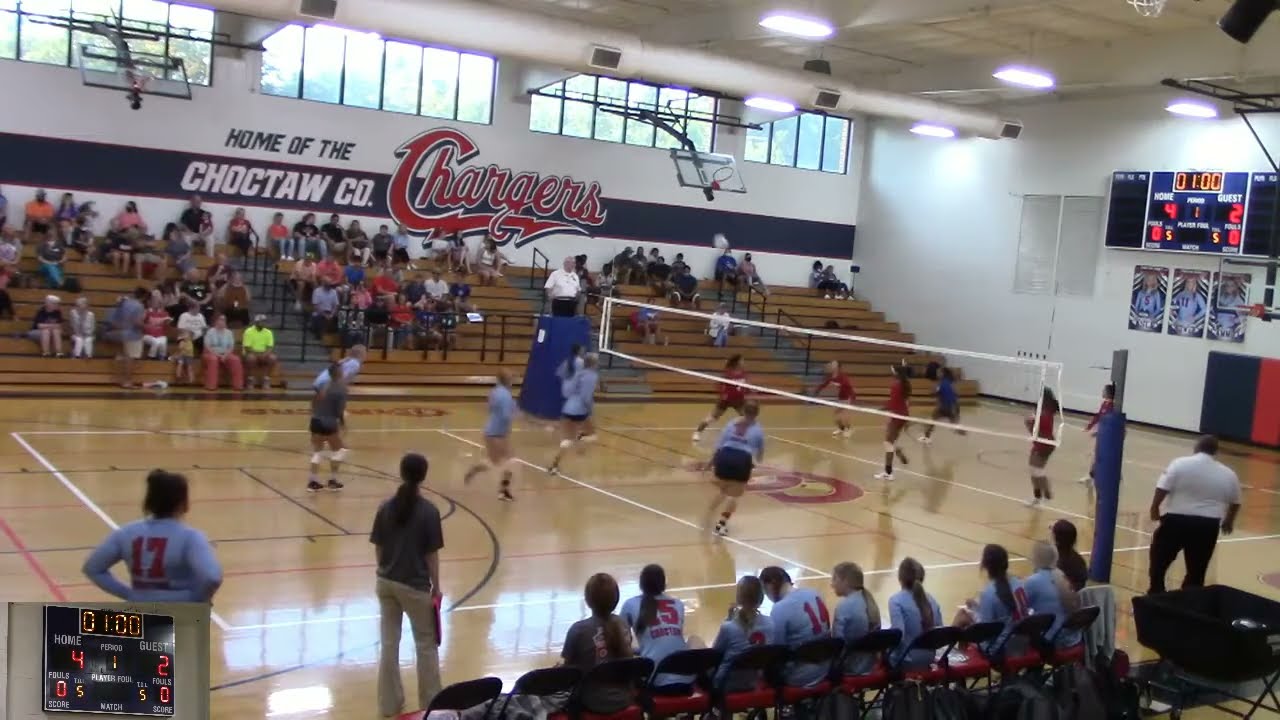This photograph, taken inside a high school gymnasium, captures an intense volleyball match between two teams. The gym’s back wall prominently displays a banner reading "Home of the Choctaw County Chargers," with "Choctaw County" in white and "Chargers" in red against a dark blue or black backdrop. The volleyball court features a brown floor marked with white and black lines, and a white net stretches across the center. Female players, dressed in red and gray uniforms, are energetically engaged in the game. On the right side of the image, the scoreboard shows one minute remaining, with the home team leading 4-2. The left bleachers are densely packed with spectators, while the right side is less populated. At the bottom left, in front of a row of foldable chairs occupied by the gray-uniformed team, a coach in khaki pants and a black shirt stands out. One player, number 17, is particularly notable. Two referees oversee the game, one perched on a stand beside the net.